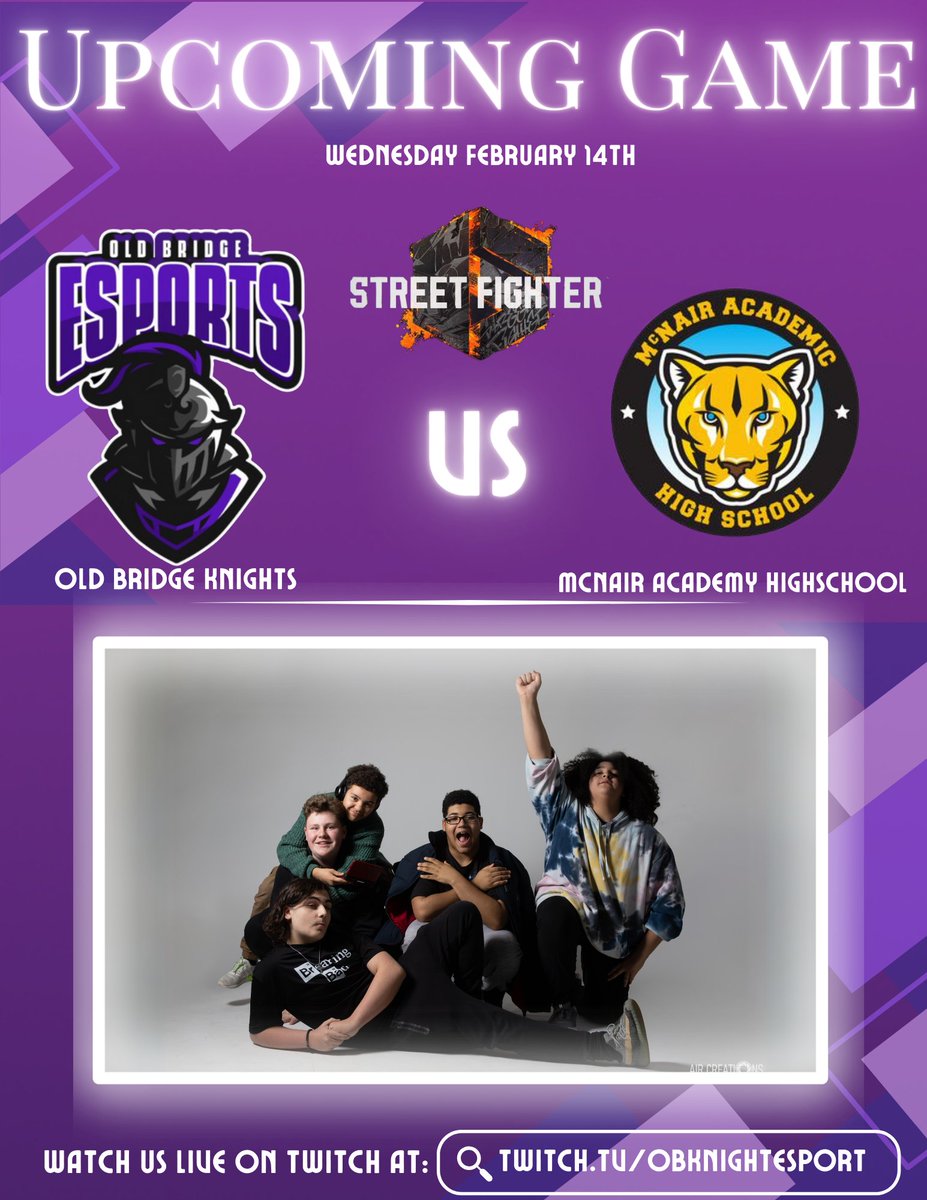This image is a detailed screenshot of a flyer for an upcoming video game competition, set against a predominantly purple background with varying shades. At the top, bold white text announces "Upcoming Game" followed by "Wednesday, February 14th." The centerpiece features a dynamic shield with fire and the title "Street Fighter." On the left, the Old Bridge Esports logo showcases a knight in shining gray armor with a blue plume and collar, underlined by the name "Old Bridge Knights." Opposing them is McNair Academic High School, represented by a mountain lion with blue eyes. Below the logos, vivid white text juxtaposes the words “V.S.” between the teams. A photo of five team members with one player triumphantly raising their fist is positioned underneath, creating a sense of camaraderie. Additionally, a call to action at the bottom of the image invites viewers to "Watch us live on Twitch at twitch.tv/obknightesport."